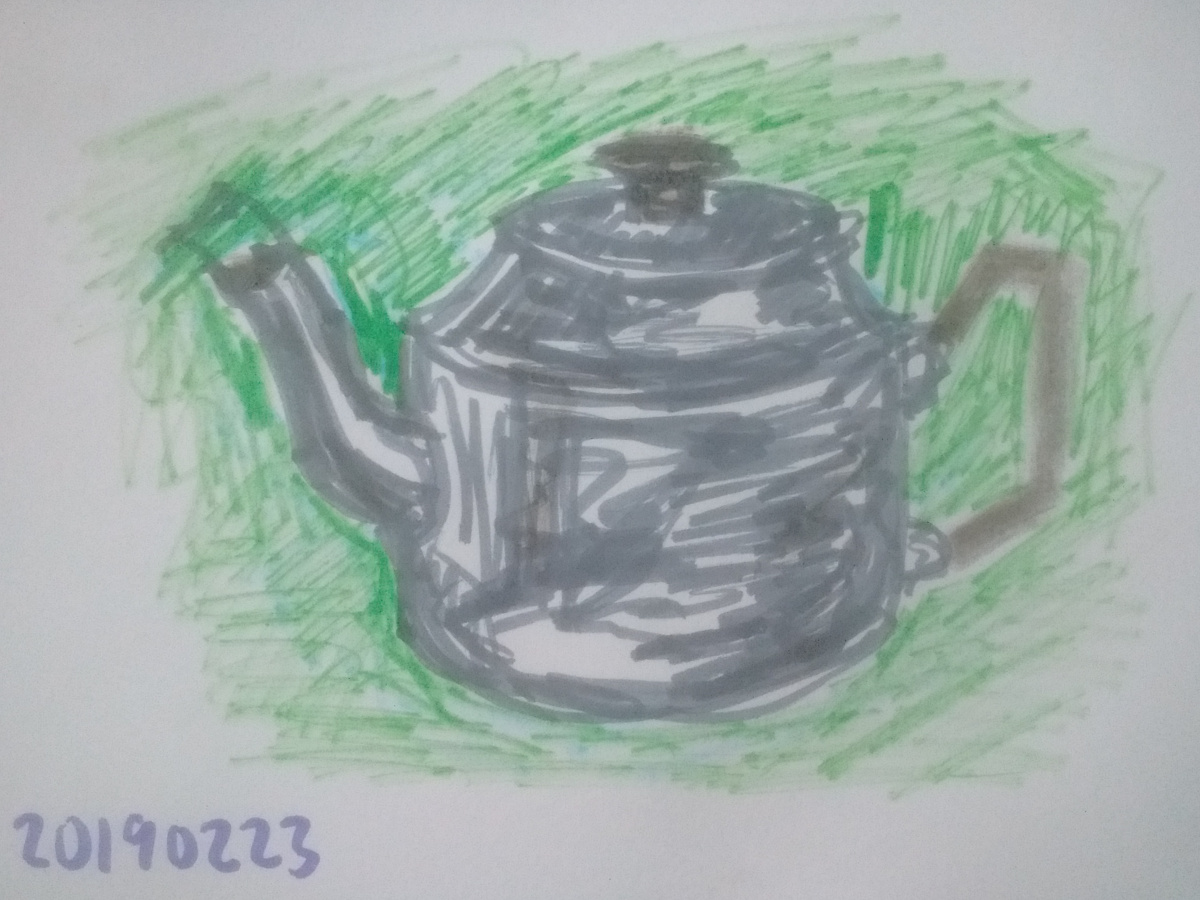The image depicts a charming child’s drawing created with markers. The drawing features a whimsical grey teapot or kettle, designed to resemble an elephant, with an elongated spout that mimics an elephant's trunk. The teapot also includes a functional-looking handle and a lid with a black knob on top. In the background, there is a simple green grassy field, adding a touch of nature to the scene. Below the teapot, a date, "2019-02-23," is inscribed, likely indicating when the artwork was created. The overall composition is straightforward and reminiscent of a standard household teapot, but the elephant motif adds a playful and imaginative twist.